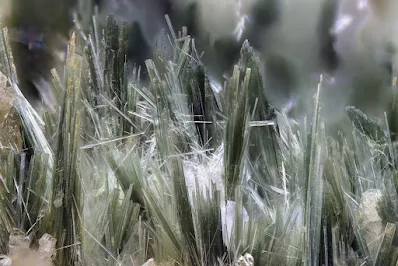The image is a highly detailed, zoomed-in close-up of a plant showcasing intricate textures and colors that make it appear somewhat ambiguous. The primary focus is on dark green, grass-like blades with fibers or protrusions visible on each leaf. There are also white patches in the middle of the image, possibly due to light hitting the plant or additional fibers. The background is blurred out, drawing attention to the sharply focused foreground. At the base, a touch of dirt is visible, adding to the natural setting. The overall color palette consists predominantly of dark green, with hints of gray and white blending in, creating a visually striking composition.